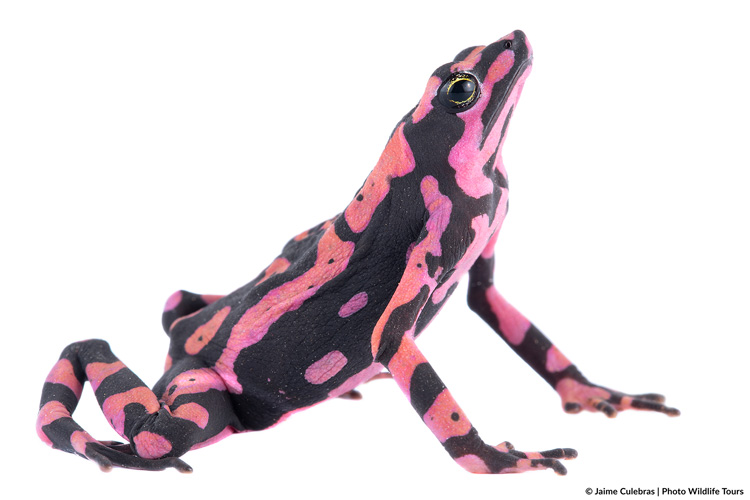This striking photograph showcases a uniquely marked, pink and black frog in a captivating, almost yoga-like pose. The frog is positioned on an all-white background, allowing its vibrant colors to stand out vividly. In the image, the frog is centered and adopting a pose reminiscent of "downward dog" with its front legs firmly planted on the ground and its back legs tucked under its body. Its head is lifted and angled upwards, giving the impression it is gazing at the sky, with its oblong black pupils surrounded by a flecked gold iris looking directly into the camera. The pink and black markings on its body are irregular, almost tiger-like, adding to its exotic appearance. Additionally, the frog's chest is primarily pink, adorned with black stripes, while its legs exhibit black and white striping, and its fingers are predominantly black. In the bottom right corner of the photograph, the credit "© Jamie Culbriss Photo Wildlife Tours" is displayed, indicating its professional and potentially promotional use for wildlife tours.